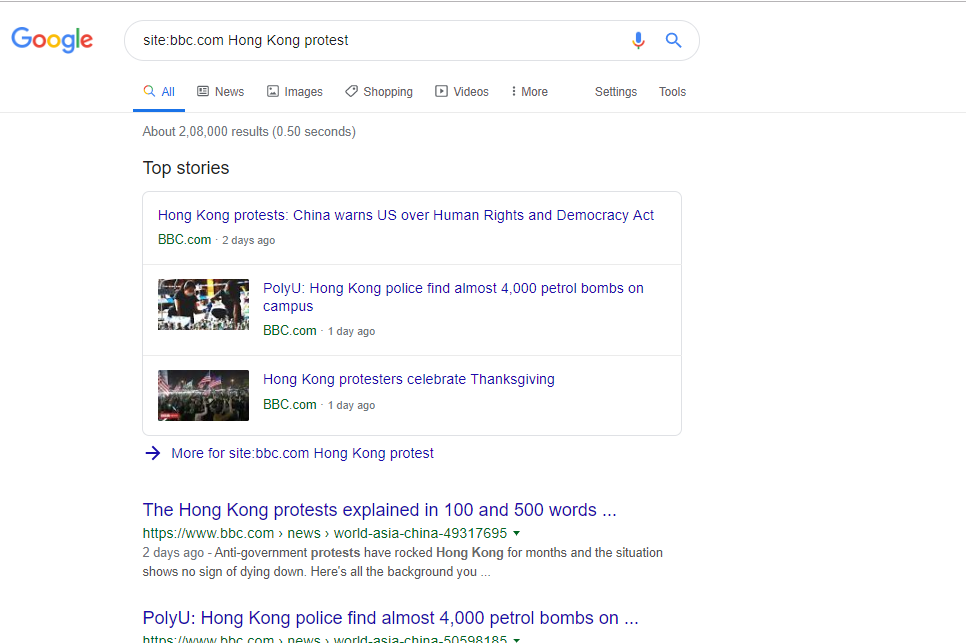The image depicts search results on Google. In the upper left corner, the Google logo is prominent, with the search bar positioned to the right. The search query entered is "site:bbc.com Hong Kong protest." Directly below the search bar, several categories are visible, with "All" highlighted in blue, indicating the active category. The other categories—News, Images, Shopping, Videos, More, Settings, and Tools—are displayed in grey, listed from left to right.

The results indicate approximately 2,800,000 hits. The "Top stories" section is prominently featured. The top result is a news article titled "Hong Kong protest: China warns US over human rights and democracy act," published by bbc.com two days ago. In this section, article titles are in blue, while the website names are in green.

Following are more results:
1. "PolyU: Hong Kong police find almost 4,000 petrol bombs on campus."
2. "Hong Kong protesters celebrate Thanksgiving."

Both of these headlines are also from bbc.com.

An arrow pointing to the right indicates additional results under "More for site:bbc.com Hong Kong protest." Two more search results are shown:
1. "The Hong Kong protest explained in 100 and 500 words" with the green website link and timestamp from two days ago.
2. A truncated result: "PolyU: Hong Kong police find almost 4,000 petrol bombs on…"

The entire display is set against a white background.